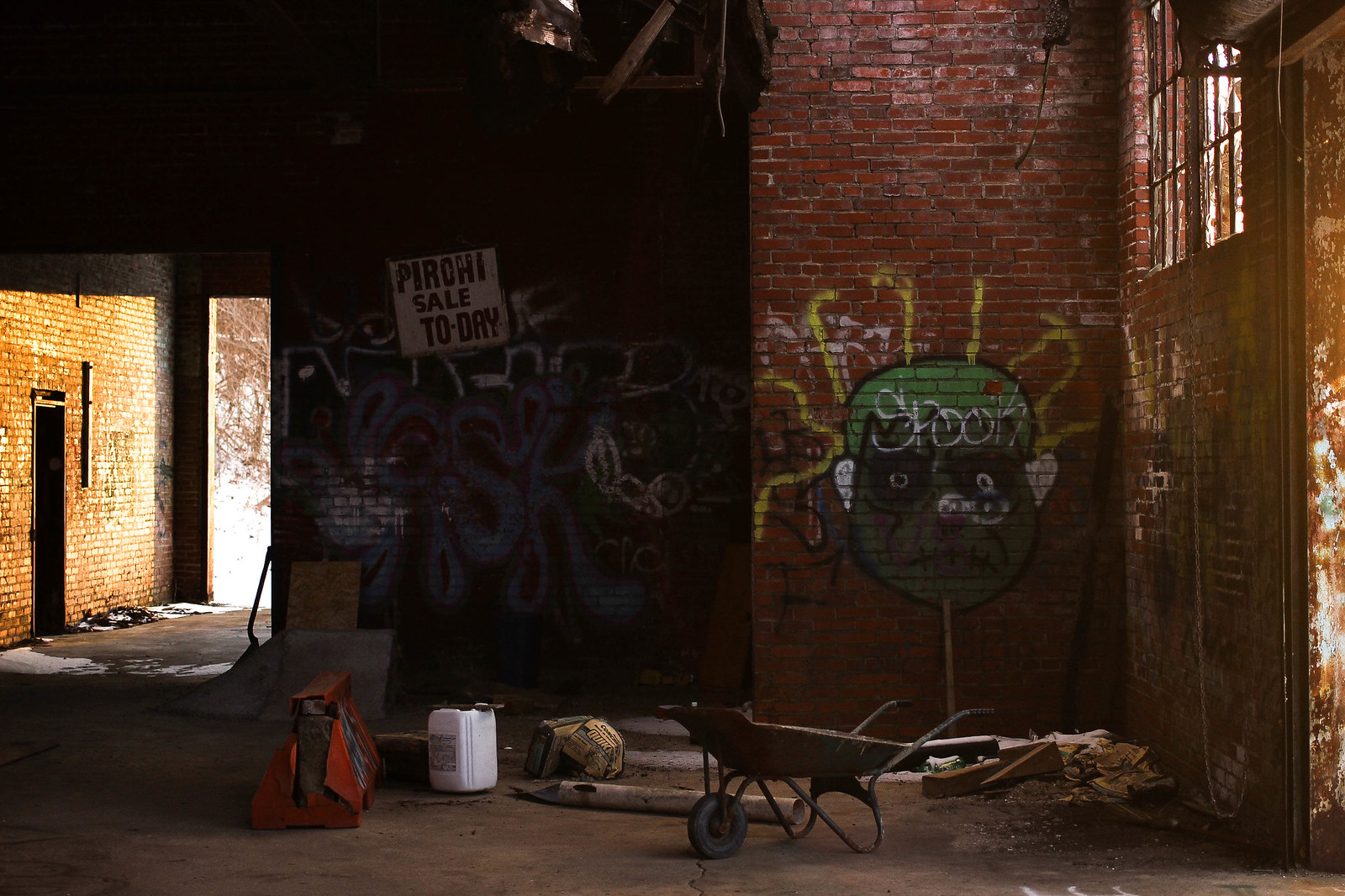The image captures the interior of an abandoned or decrepit brick building, likely a warehouse or industrial space, with multiple red brick walls set at different angles. Graffiti adorns these walls, including a notable image of what looks like a green-faced character with yellow hair streaming out, possibly resembling Medusa or an alien. On one of the walls, there's a spray-painted sign in blue letters reading "Pirohi Sale Today" or a similarly misspelled version of "Pierogi Sale Today" amidst other graffiti.

The room is cluttered and dirty, featuring scattered construction tools such as a wheelbarrow, a gasoline container, and a large bag on the cement floor. Daylight streams through a large, doorless opening on the left side, illuminating the messy space. This opening leads to another part of the building in the distance, where a distant wall has two small windows, hinting at more enclosed spaces further inside. The overall impression is of a space that's either abandoned or staged to appear neglected, with debris and urban artwork adding to the sense of disarray and abandonment.